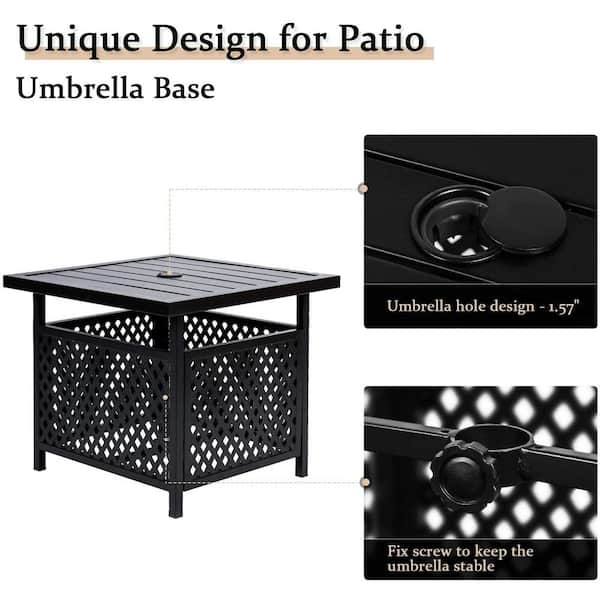This advertisement presents a unique patio umbrella base in a clean, white background. At the top, the text "Unique Design for Patio" is displayed in black letters, underlined by a tan rectangle spanning the width of the image, followed by the words "umbrella base". The central focus is a black metal table with a slatted top and four sturdy legs. The table features a central hole with a metal lattice surrounding the table's underside, giving the appearance of a basket-like structure. Two inset images provide a closer look at specific features: the first shows the umbrella hole design with a measurement of 1.57 inches, while the second highlights a screw system, labeled "fix screw to keep the umbrella stable," designed to secure the umbrella in place.